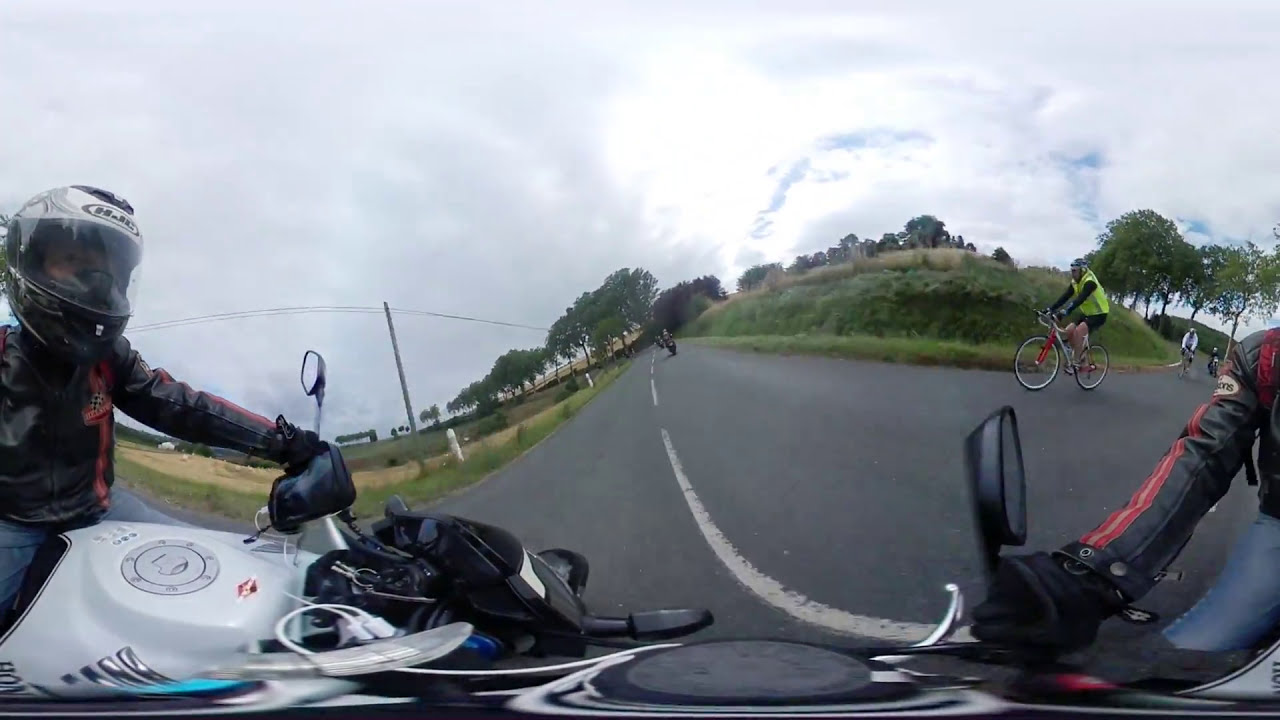This outdoor image appears to be captured by a GoPro or helmet-mounted camera of a motorcycle rider on a wavy, two-lane road. The sky is overcast with gray clouds, and hills undulate in the background, covered in greenery and trees. In the foreground on the left, a motorcyclist rides a white motorcycle, and is dressed in a black and red jacket, black and white helmet, and gloves. Only the arm of another motorcyclist, clad in black leather with a red stripe, is visible to his right. Ahead, a bicyclist wearing a green safety vest, black long-sleeve shirt, and shorts can be seen. Further along the road, other riders – some on bicycles and possibly motorcycles – are visible, including one in white. Behind this scene, additional trees and power lines are visible, adding depth to the image. The fisheye lens perspective gives the photo an extreme, curved effect.